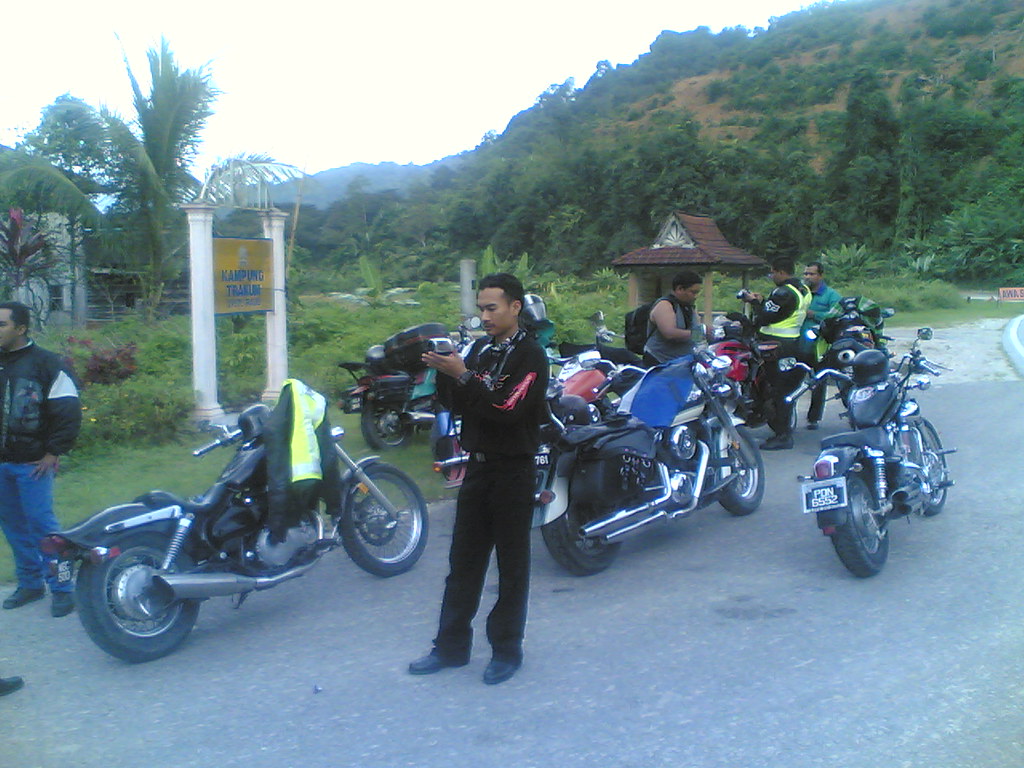In this detailed color photograph, a group of motorcycles is lined up along a concrete asphalt path on the outskirts of a park, all facing away toward the horizon. A man dressed in all black with a red stripe down his long-sleeved shirt stands in the center, holding a camera and directing it toward the left side of the image. He has dark hair and skin. Nearby, two other men in dark jackets and blue jeans are partially visible, engaged in conversation. The motorcycle closest to the camera is black with a yellow and white jacket draped over its handlebar. In the background, an overcast sky casts a muted light over the scene, which includes a grassy area, palm trees, and a hill covered in trees and green shrubs. In the distance, a park sign mounted on two white columns with gold and blue lettering, stating "Camping Trailer," is visible. There is also a small structure with a brown shingle roof, possibly for ticketing, adding to the realistic and representational style of the image.